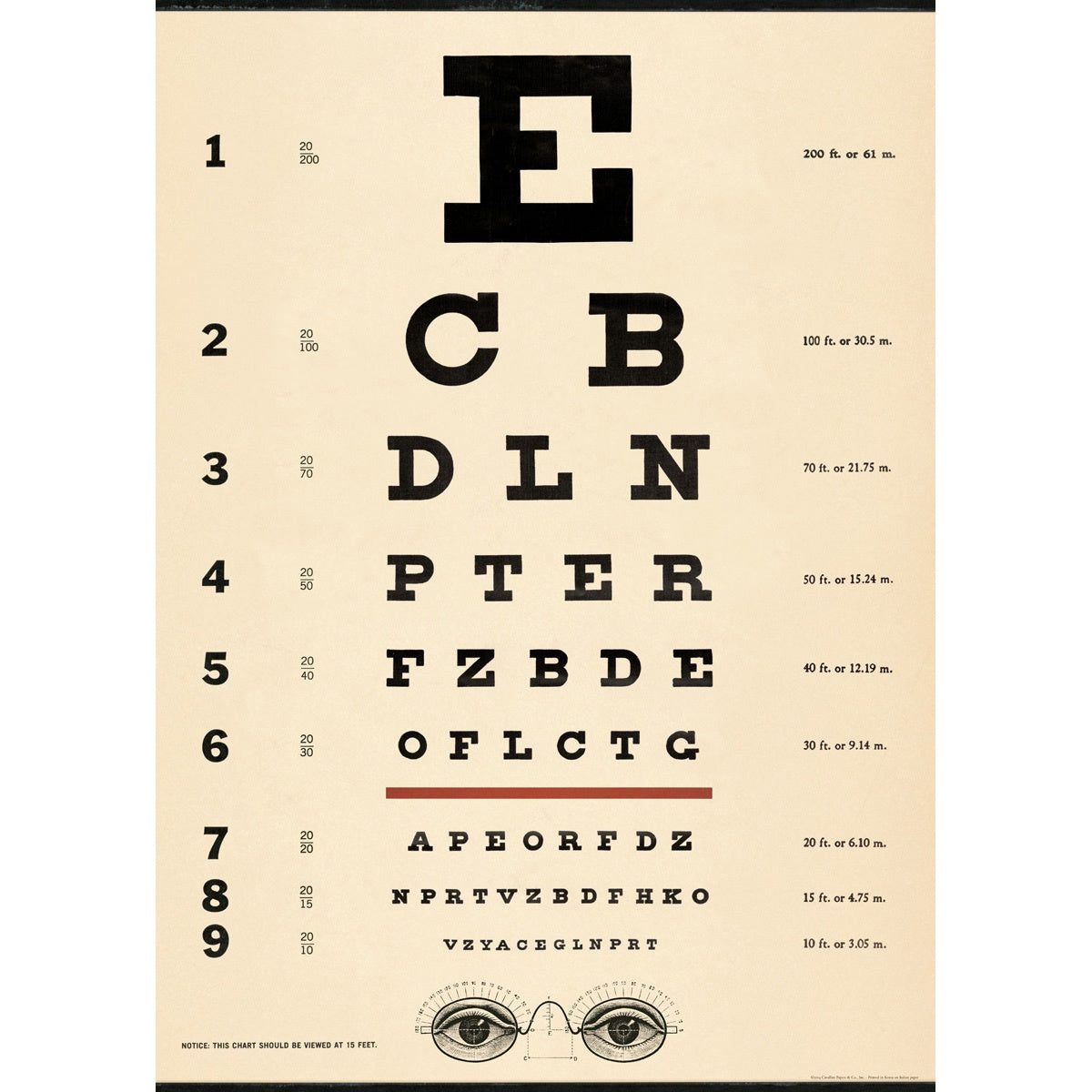The image depicts a vintage eye test chart designed to measure visual acuity in both feet and meters. The chart is beige with a black border at the top and bottom. It features nine rows of capital letters that progressively decrease in size from the top to the bottom. The first row begins with a large "E" labeled as "20/200" (200 feet or 61 meters), followed by "CB" on the second row marked "20/100" (100 feet or 30.5 meters), and continues with "DLN" on the third row labeled "20/70". Each subsequent row contains more letters that grow progressively smaller. By row seven, which marks the "20/20" vision level, this classic eye chart serves as a tool for optometrists to determine the necessity and strength of corrective lenses. At the bottom of the chart, there’s an illustration of a pair of glasses and an additional image of two eyeballs, likely indicating further details used in the diagnostic process. The vintage aesthetic underscores the traditional method of eyesight testing employed in the past.